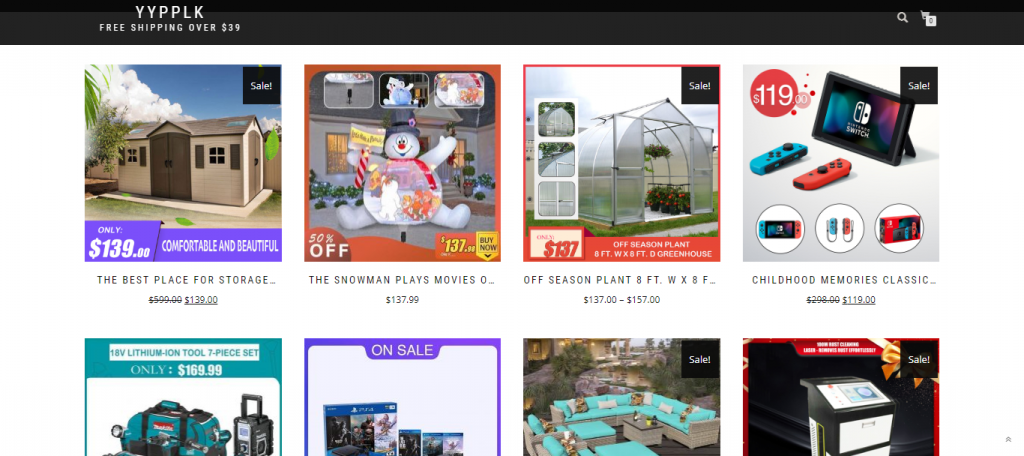In this image of a website, various items are displayed for sale, each accompanied by thumbnails and item descriptions. At the top of the webpage, a black horizontal border features the text "YYPPLK" in white font, along with a notice for "free shipping over $39." On the right side of this border, there is a search icon, represented by a magnifying glass, followed by a shopping cart icon with the number zero, indicating that no items have been added to the cart yet.

Beneath this header, several items are showcased:
1. A storage shed is advertised as "The best place for storage" priced at $139.00, described as "comfortable and beautiful."
2. An inflatable Christmas decoration of a snowman titled "A snowman plays movies," priced at $137.99.
3. An off-season plant item described as "8 foot, with X8F" priced at $137.57, showing a greenhouse filled with red flowers.
4. A Nintendo Switch is listed under "Childhood memories classic" for $119.00.
5. A seven-piece tool set image follows, though without additional details or price mentioned.
6. A PlayStation 4 is included, presumably for sale.
7. An outdoor sectional seating arrangement, consisting of a sectional chair, ottomans, and a table with cushions in a neon blue (or teal/aquamarine shade).
8. Finally, a printer is displayed in the bottom right corner.

This detailed layout provides a diverse range of products from storage solutions to holiday decorations, gaming consoles, outdoor furniture, and electronics, appealing to a wide array of interests and needs.